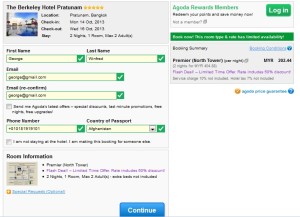The web page appears to display information about the Berkeley Hotel, which seems to be located in a city starting with the letter 'P,' potentially in Bangkok. The header section in the upper left corner features the hotel’s name, "Berkeley Hotel," and a blurred, small-font text specifying the city's name. Beneath the hotel name, a photograph presumably showcases the hotel's exterior, highlighting a clear blue sky and what appears to be a swimming pool, all set against a light blue background.

The middle section of the page contains input fields for user information, arranged in several boxes. These fields are labeled for first name, last name, email, an additional email confirmation, phone number, and country of passport, allowing users to select and fill in their respective details.

Towards the bottom of the page, there is a segment with two discernible words in black text, with the latter word being "information." This section likely provides further contextual or detailed information about the hotel.